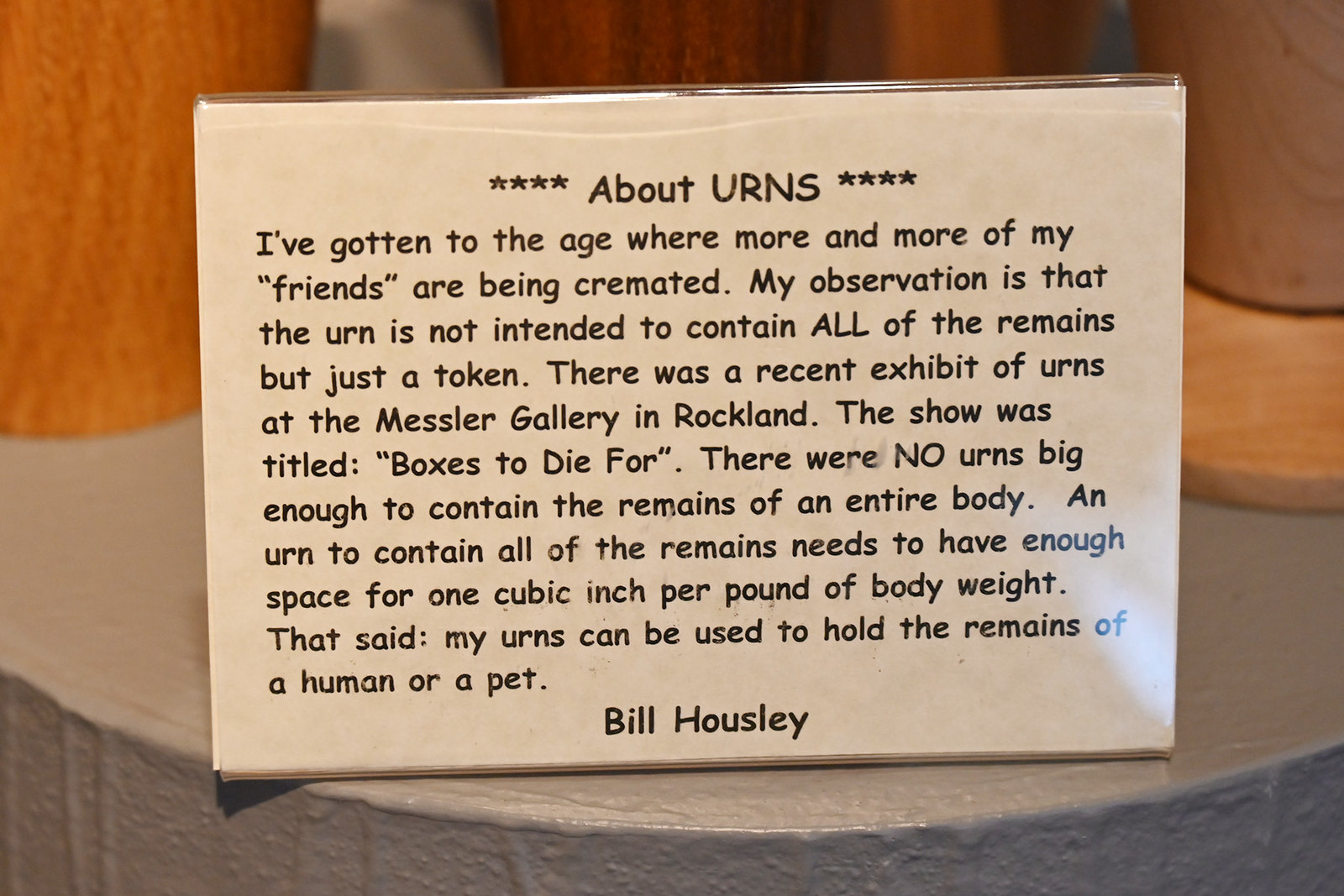This landscape-mode photograph captures a somber scene inside a funeral parlor. Central to the image is a prominently displayed message encased in plastic, written by a person named Bill Housley. The sign is titled "About Urns," with four asterisks flanking both sides of the title. Below the title, the text explains Housley's observations on cremation urns, noting that they are often not intended to contain the entirety of a person's remains, but rather a token amount. Housley mentions a recent exhibit of urns at the Messler Gallery in Rockland titled "Boxes to Die For," and explains that no urns there were large enough to hold all of a body's ashes, which would require one cubic inch of space per pound of body weight. He concludes by stating that his urns can hold the remains of either a human or a pet.

The sign sits atop a grey-painted countertop or plinth. In the background, partially visible, are several wooden urns of varying shades of brown, arranged across the top of the grey surface. The overall tone of the image is muted, aligning with the somber subject matter, and the text appears to be in Comic Sans font, enhancing the personal, handwritten feel of the message.